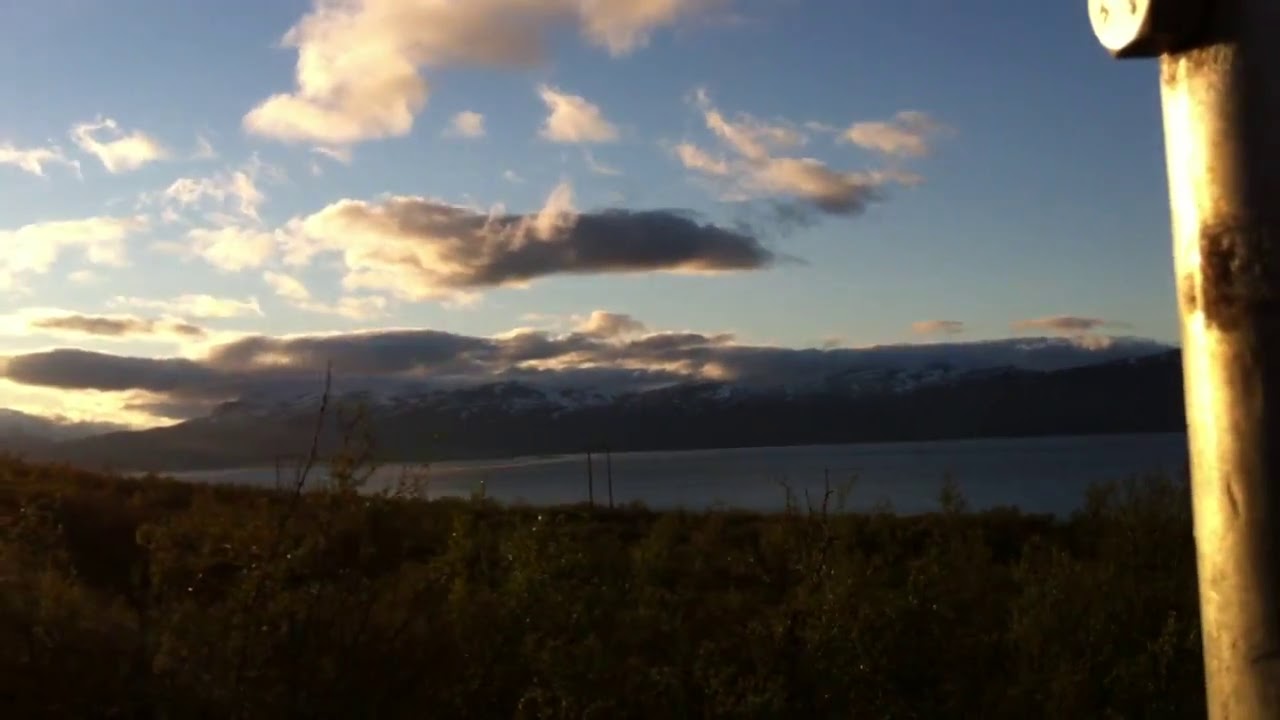This detailed landscape photograph captures an outdoor natural setting at either evening or dusk. In the foreground, there is a grassy ground populated with brownish weeds and green plants. Moving towards the middle of the image, a large body of water, possibly a lake or a river, spans the entire width of the photograph, its surface reflecting the diminishing light of sunset. Beyond this water body, the horizon features a range of mountains with their snowy peaks visible, suggesting higher elevations. The sky above these mountains is a dynamic blend of blue hues with various clouds, ranging from dark, dense formations to lighter, fluffy ones, all illuminated by the subtle, golden rays of the setting sun. On the right side of the image stands a vertically positioned wooden log or post, its brown surface gleaming with a golden sheen from the sunlight. The serene yet dramatic contrast between the natural elements creates a captivating scenic view.